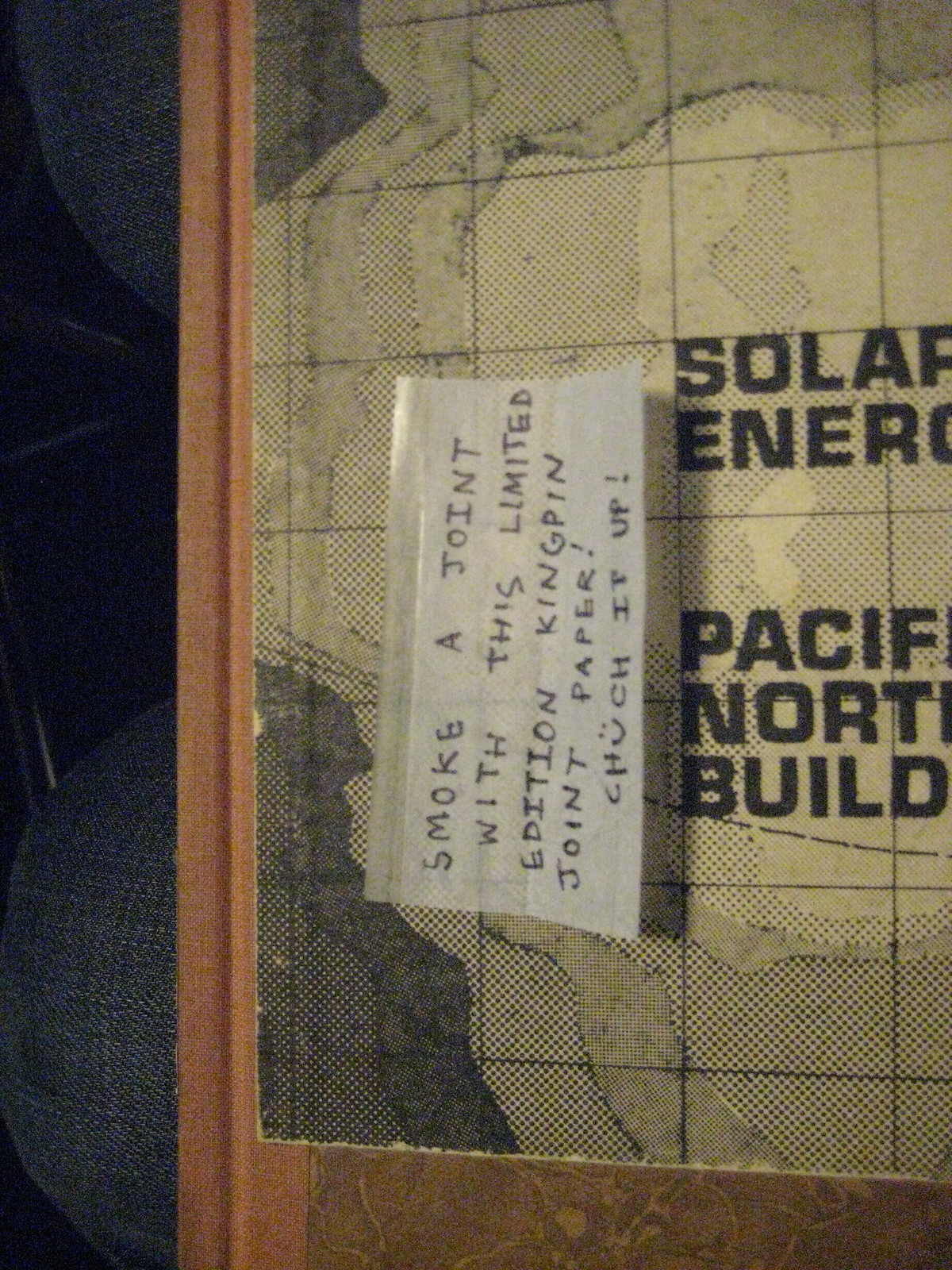This image appears to capture a laminated, detailed map or photo related to solar energy in the Pacific region. Affixed to this map is a white piece of paper hanging downwards, also laminated, with text that is not completely legible. The visible words on the paper mention "Solar Energy," "Pacific," and "North," suggesting it details a solar energy project or network in the Pacific Northwest. The color palette of the map includes shades of brown, off-white, and black. The paper attached seems to be hanging loosely and slightly tilted, with its text oriented from left to right towards the top. The overall setting of the photograph remains ambiguous—it is unclear whether it was taken indoors or outdoors. The surroundings and detailed contents of the map/photo contribute to the context but are not completely discernable due to the angle and positioning.